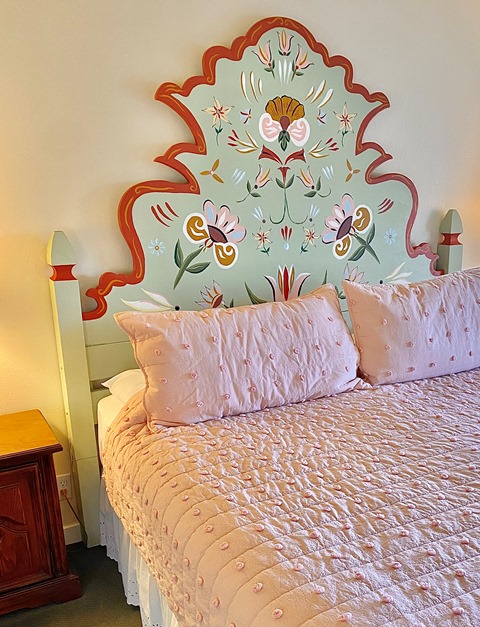This image captures a sumptuous hotel room or bedroom, dominated by a grandiose bed set against a light cream-colored wall. The headboard is a standout feature—it's a large and intricately designed piece with a curvaceous, rounded shape, flanked by wooden columns that rise up and culminate in triangular caps. The headboard itself is primarily light green, adorned with a vibrant painting of a mixed bouquet of flowers in various shades of pink, green leaves, and interspersed hues of yellow, white, purple, and light blue. At the top center of the headboard, a large flower is prominently displayed, flanked by two equally large flowers on either side, with more flowers scattered around them in a lively pastel green background.

The bed is dressed in a coordinated set of pink comforter and pink pillowcases, under which white sheets peek out, adding a crisp contrast to the rich colors of the floral arrangements. The white sheets extend all the way down to the floor. Positioned beside the bed, to its left, stands a modest brown wooden nightstand, about two to two and a half feet tall, adding a functional yet unobtrusive touch to the luxurious setting.